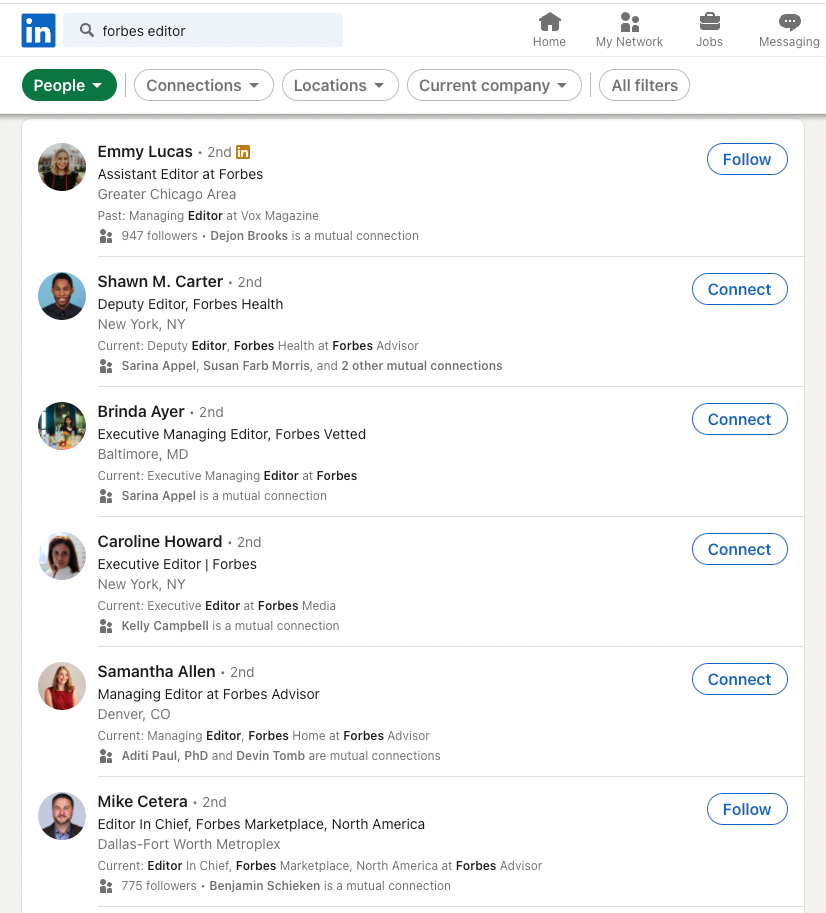Certainly! Here is a cleaned-up and detailed caption based on the voice description:

---

The image features a user interface from a job search platform. At the top left, there is the Indeed logo prominently displayed with the letters "I," "N," and "white" on a blue square. Adjacent to the logo is a search bar with the text "Forbes editor" entered. 

To the right of the search bar, the navigation menu includes the following options from left to right: "Home," "My Network," "Jobs," and "Messaging." Below the navigation bar, there is a set of filter options starting with a green pull-down menu on the left with white text. Next to it, there are various pull-down options with white backgrounds, gray outlines, and gray text: "Connections," "Locations," "Current Company," followed by "All filters."

The primary content section beneath this navigation is on a white background and lists three professional profiles:

1. **Emmy Lucas**
   - Featured within a white box with an orange "I, N" icon.
   - Title: Assistant Editor at Forbes, located in the Greater Chicago Area.
   - Past Role: Manager, Editor at Vox Magazine.
   - Additional Info: Emmy has 947 followers with one mutual contact, Dijon Brooks.
   - There is a "Follow" button on the right side.

2. **Sean M. Carter**
   - Profile within a similar white box.
   - Title: Deputy Editor, Forbes Health, located in New York, New York.
   - Current Role: Deputy Editor, Forbes Health at Forbes Advisor.
   - Mutual Contacts: Saren Akhil, Susan Barb Norris, and two others.
   - Contains a "Follow" button on the right side.

3. **Brenda**
   - The profile content begins below Sean M. Carter, though additional details are truncated in the description.

The backdrop remains consistently white, enhancing readability and a clean user experience.

---

This caption provides a comprehensive and clear description of the image as described in the voice note.